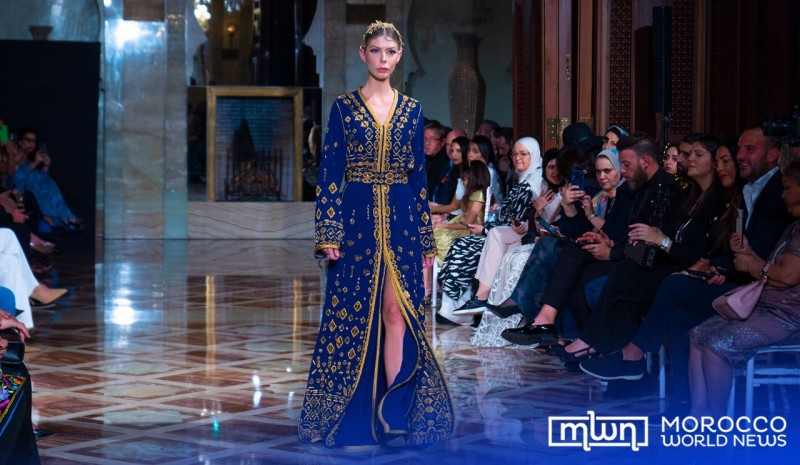In this landscape photo, a fair-skinned model walks down a tiled runway, centered in the image. She is wearing a striking blue gown with intricate yellow accents, split in the middle to reveal her left leg, ensuring ease of movement. Her light brown hair is sleekly parted down the middle and pulled tightly back, highlighting her confident posture. The runway is lined with spectators on both sides, with more attention from those on the right, some engrossed in their phones while others are captivated by the show. The scene is set in a dimly lit room, making the well-lit model the focal point. The glossy runway reflects the lights, adding to the glamor of the event. Text on the bottom right corner reads "MWN" with "Morocco World News" slightly further to the right against a semi-transparent blue background, confirming the prestige of the occasion.